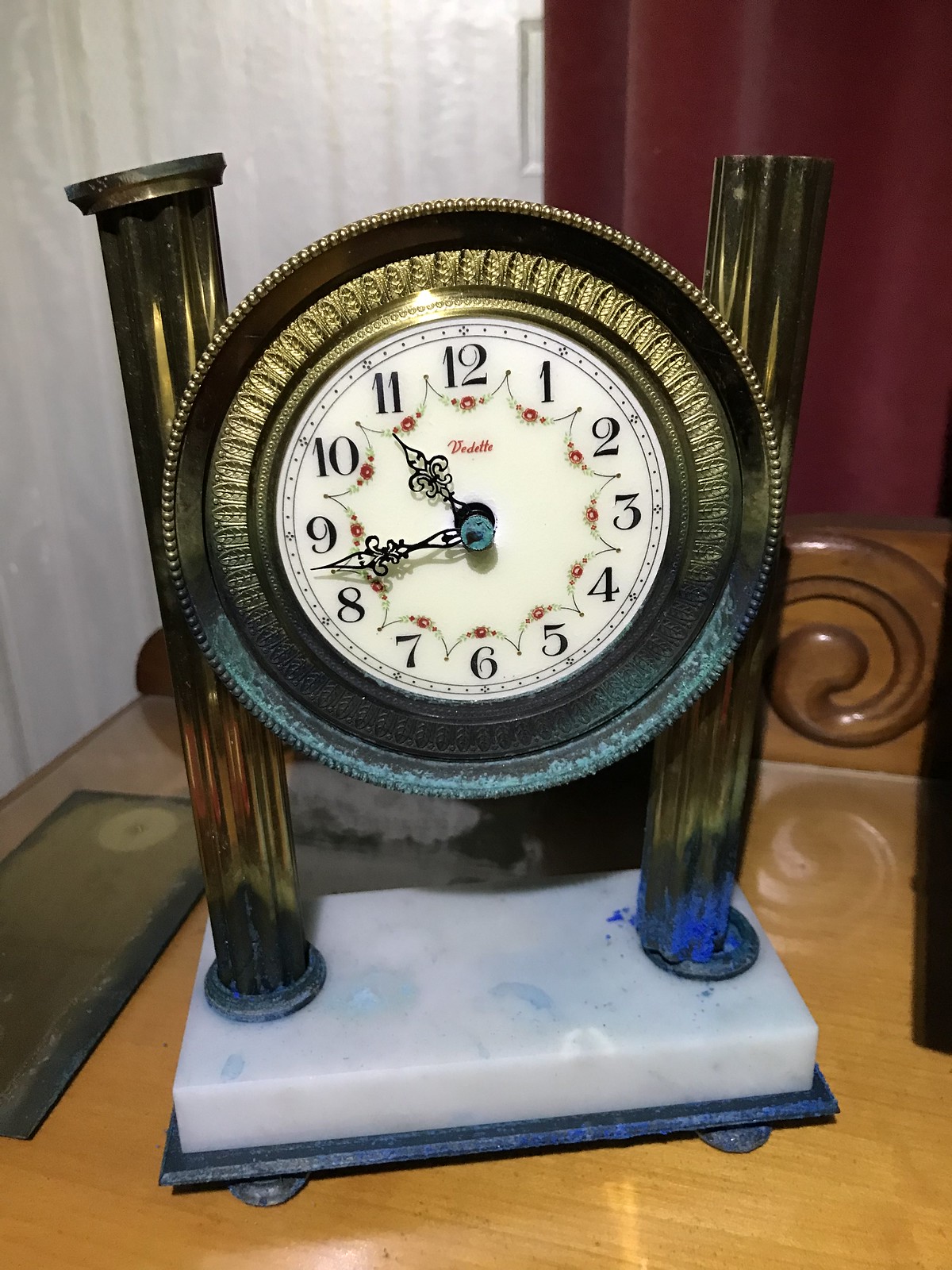This image features a meticulously designed clock that bridges past and futuristic aesthetics. The clock is encased within a bronze plate, which is prominently situated between two vertically standing bronze bars. These bronze bars are anchored into a sturdy granite base with a white upper section and a gray lower section, reminiscent of a trophy pedestal. The base itself stands on two legs, providing stability and an elegant elevation. The clock face is classic white, adorned with black numerals from 1 through 12, and the clock hands indicate the time is 11:45. This timepiece serves as a symbolic blend of historical craftsmanship and forward-looking design.